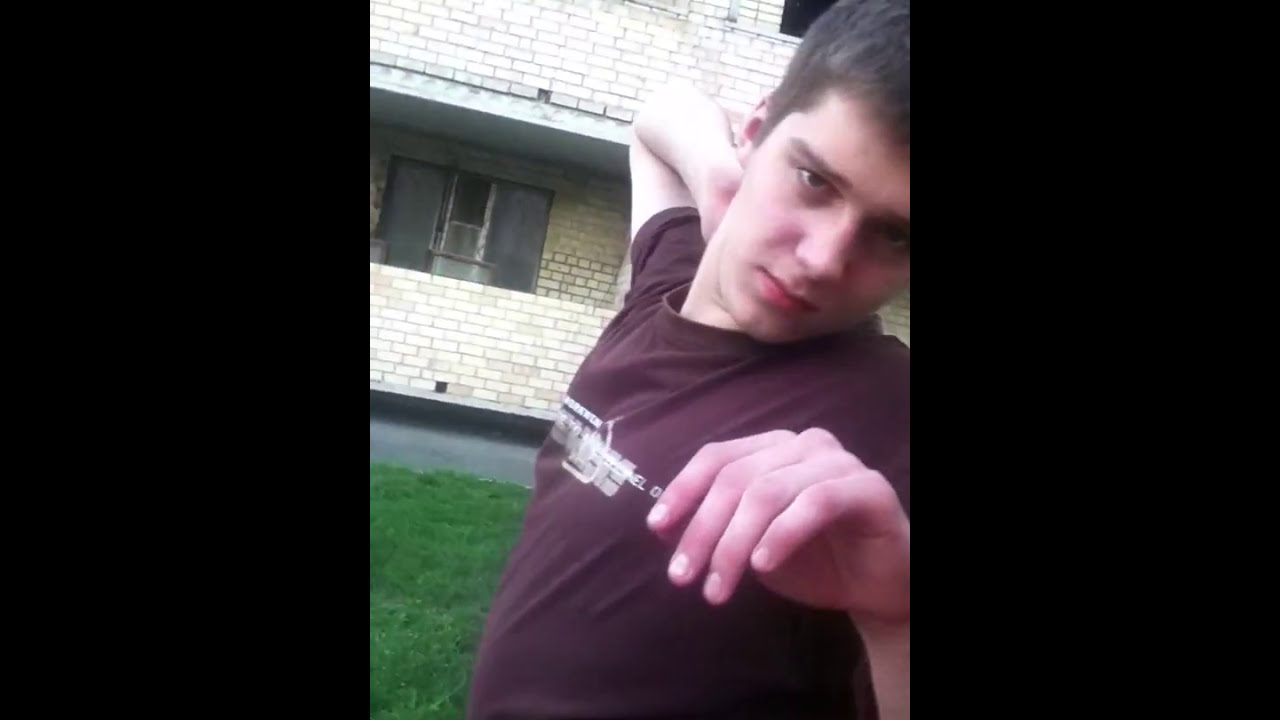The image is a horizontally aligned rectangular photograph surrounded by thick black borders on the left and right sides. The central, dominant panel of the image features a young man, appearing to be in his late teens to early twenties. He has short brown hair and is wearing a short-sleeve brown or dark red t-shirt with an indeterminate white text and graphic design across the chest. The man's pose suggests he is stretching or possibly yawning; his right arm is bent, with his hand placed at the back of his neck, while his left arm is raised and extended outward. He looks directly at the camera with a neutral expression, his mouth closed. 

Behind him, a two-story building with white and gray bricks stretches across the backdrop. The building looks old and somewhat rundown, with a weathered window visible on the lower level. The scenery includes a grassy lawn in front of the man, with a sidewalk stretching in front of the house. The lawn appears well-maintained, with the grass cut short. The contrast between the vivid, detailed central panel and the plain black borders serves to highlight the young man as the focal point of the photograph.